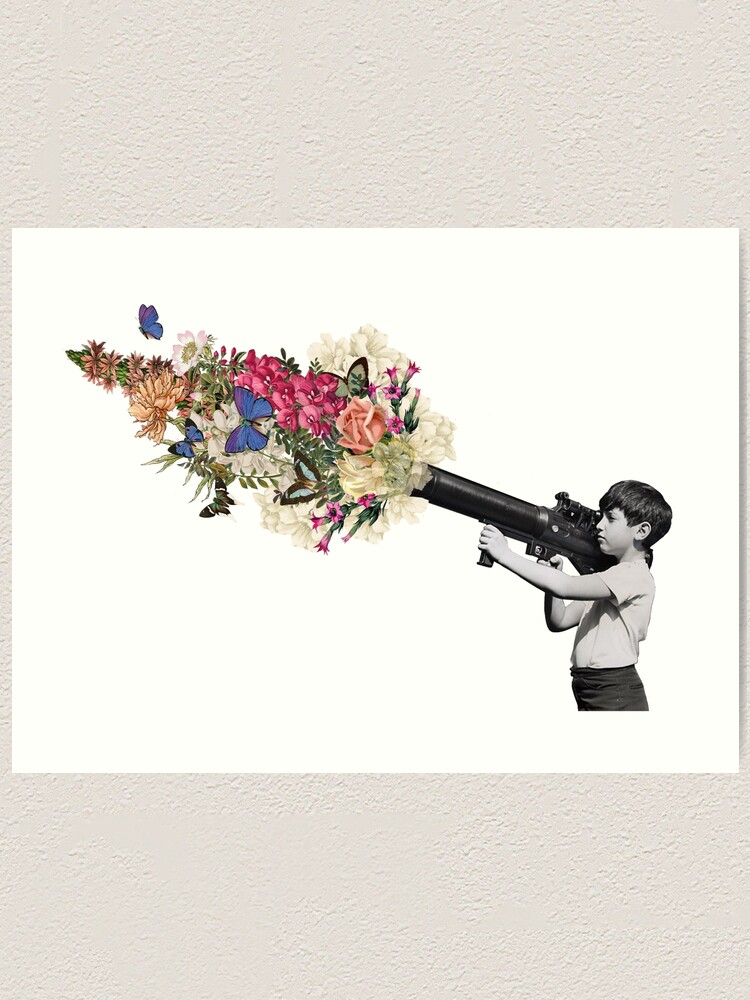In this tall rectangular artwork, set against a textured off-white and light gray painted wall, a wide beige-colored piece of paper features a compelling collage. The central image is a black-and-white cut-out of a young boy, visible from the hips up, standing near the right side of the paper and facing left. He holds a very large, long black gun on his shoulder, with one arm outstretched to hold its lever and the other gripping the trigger. The boy, with short black hair and wearing a short-sleeved shirt tucked into his pants, appears to be focused on his task. Contrasting the stark monochrome of the boy and the gun, the cannon’s barrel bursts forth with a vivid and colorful assortment of flowers, butterflies, and leaves, including pink and white flowers, blue and green butterflies, and various lush details. One butterfly flies near the top left corner of the artwork, adding a whimsical touch. The collage's playful and imaginative elements create a striking and thought-provoking visual contrast.